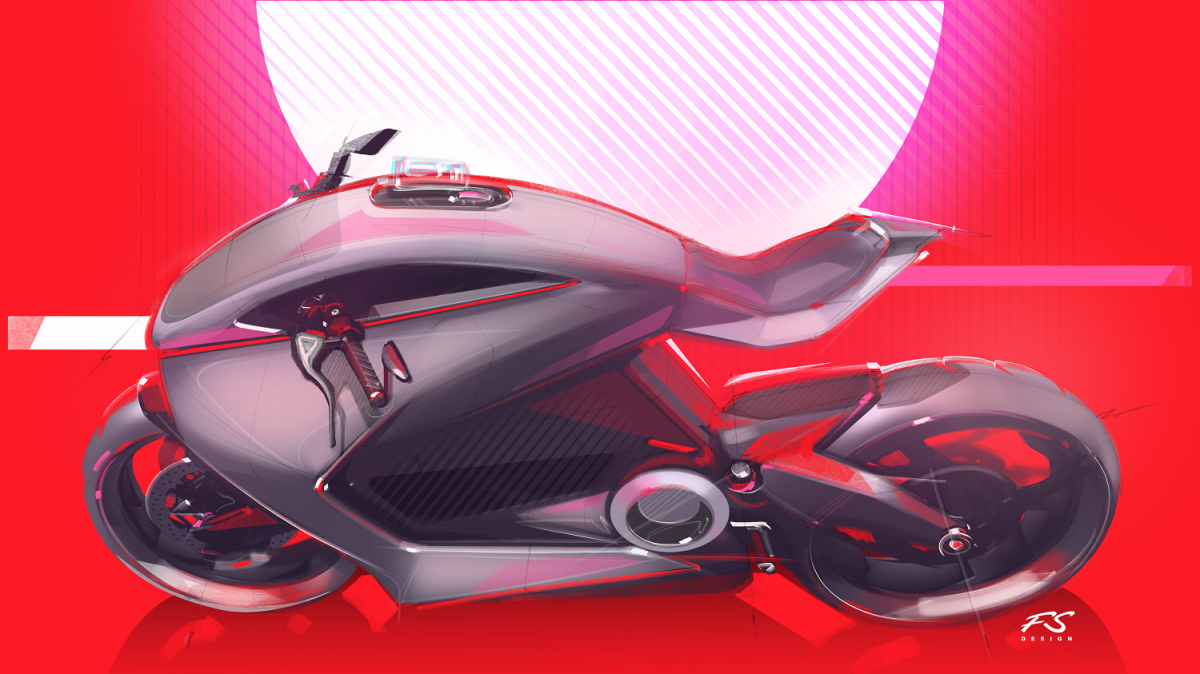This detailed color illustration depicts a futuristic motorcycle envisioned for the future. The scene is set against a vibrant red background, punctuated by a bold white stripe running horizontally from left to right. Above this stripe towards the center of the image, there is a large glowing white circle with intricate pink lines crosshatching through it, adding a layer of dynamism to the backdrop.

The motorcycle itself is a striking, smooth silver creation with an aerodynamic, wind tunnel-inspired design. It features a black, floating seat that extends from the front but lacks rear support, appearing to be held by a suspension arm attached to the rear wheel. The body of the motorcycle is curvy and cylindrical, with a bulbous front tapering towards the back. The gleaming surface is adorned with sleek red stripes, enhancing its modern and futuristic aesthetic.

The handle grips protrude from within the motorcycle's integrated tank cover, suggesting a streamlined control system that includes possible pop-up holographic interfaces or a slot for mobile device docking. Additionally, very faint continuous lines throughout the image indicate that this was originally a sketch that was meticulously colored in and refined, adding to its concept art allure. In the bottom right corner, there is a barely legible logo featuring the letters "FS" over an illegible line of text. Overall, the illustration combines vivid background elements and intricate design details to present a highly futuristic and eye-catching motorcycle concept.